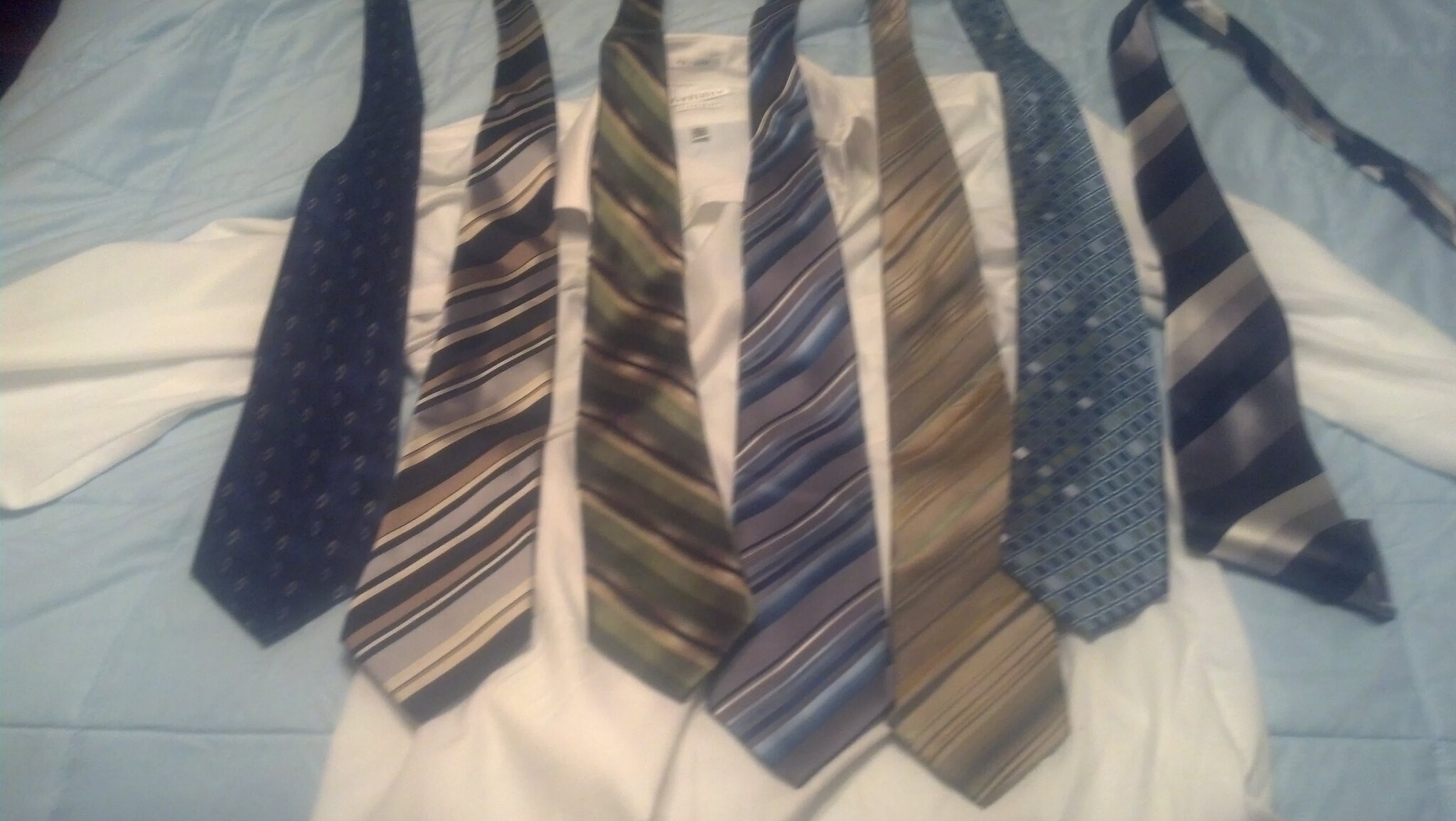This is a blurry color photograph featuring a white button-down shirt laid flat on a light blue surface, possibly a bed quilt or comforter, with the arms splayed out. Arranged on top of the shirt are seven neckties of various patterns and colors. Most of the ties feature shades of blue, brown, and yellow. Specific designs include a navy tie with dark patterns, a tan tie with black and light blue diagonal stripes, a green tie with maroon and lighter green stripes, a blue tie with maroon and gray stripes, a light brown tie with stripes, a blue tie with light blue and navy polka dots, and a black, gray, and white striped tie. The image appears shadowy and blurry, emphasizing the different colors and patterns of the ties against the crisp white shirt.